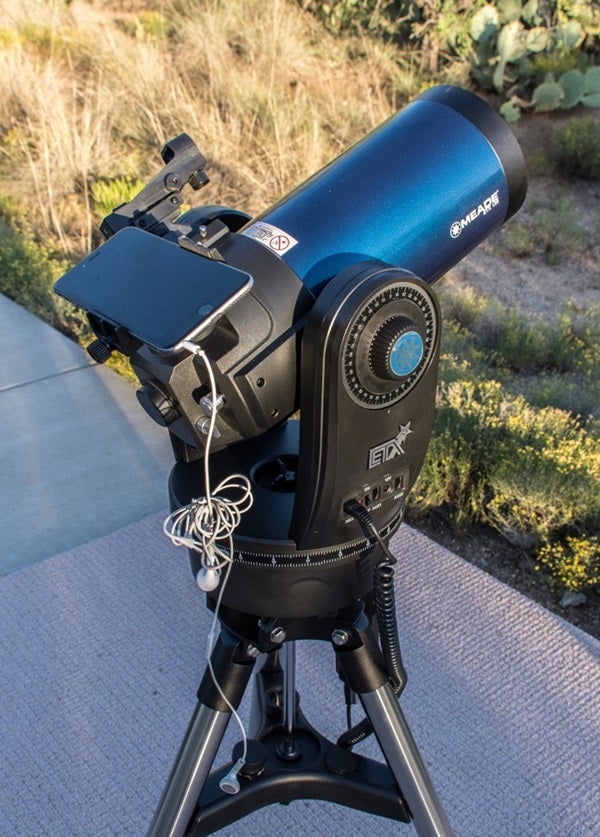The image captures a detailed outdoor scene featuring a sophisticated telescope setup amid a desert-like environment. The focal point is a blue metallic Mead telescope positioned on a sturdy black plastic ETX base. This base is affixed to a three-legged metal tripod, anchoring the ensemble on a concrete surface layered with a gray mat. A smartphone, identified as an iPhone without a case, sits perched atop the telescope, connected to a pair of tangled white corded headphones, likely Apple earbuds. The backdrop reveals an array of desert foliage, including cacti and dry grasses interspersed with green plants, suggesting a natural and arid locale.